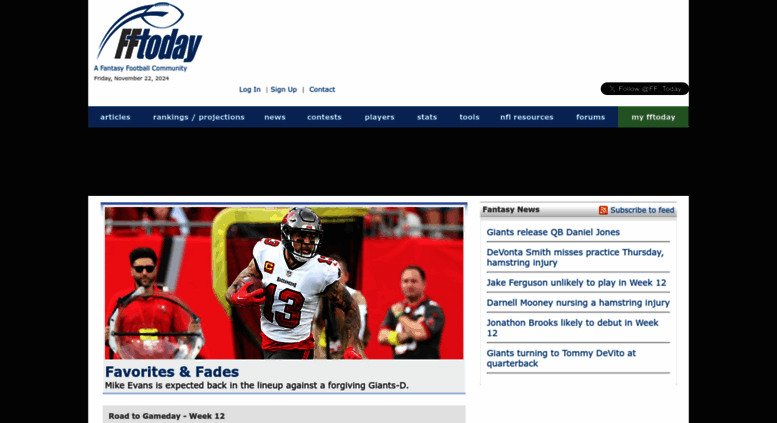The website depicted in the image is dedicated to fantasy football enthusiasts, prominently titled "FF Today," which stands for Fantasy Football Today. Located in the top left-hand corner, there is an engaging graphical logo featuring a football in flight, symbolizing the dynamic nature of the sport. The bold, eye-catching "FF Today" text is rendered in a blend of gray and blue hues, emphasizing its importance and making it easily identifiable.

Below the logo, the tagline "a fantasy football community" clearly conveys the purpose of the website, creating a welcoming atmosphere for football fans. Adjacent to the tagline are essential navigation options labeled "log in," "sign up," and "contact," allowing users to easily interact with the community. On the right-hand side, there is a like button to engage with the website's content.

The main navigation bar provides a plethora of organized sections: Articles, Rankings, Projections, News, Contests, Players, Stats, Tools, NFL Resources, and Forums. A distinctive green-highlighted section on the far right features "My FF Today," offering personalized content for registered users.

Directly beneath the navigation bar, a vivid action shot showcases a game between the Minnesota Vikings and the Philadelphia Eagles, capturing the thrill of live football. Flanking this image to the right is a list of up-to-date news headlines, including:
- Patriots extend Rhamondre Stevenson
- T. Higgins signs franchise tag
- DeJuan Johnson to undergo surgery
- Darren Waller announces retirement
- Chiefs re-sign Mecole Hardman on a one-year deal
- Vikings lock in Justin Jefferson with a four-year extension

To the left, the highlighted main article titled "The Big Uglies, NFC: Grading Out the Big Folks Up Front in the NFC" grabs attention, indicating an insightful analysis of offensive linemen performance. Below this, in smaller text, appear sections for Projections and Rankings, which are essential tools for fantasy football players to strategize and optimize their teams.